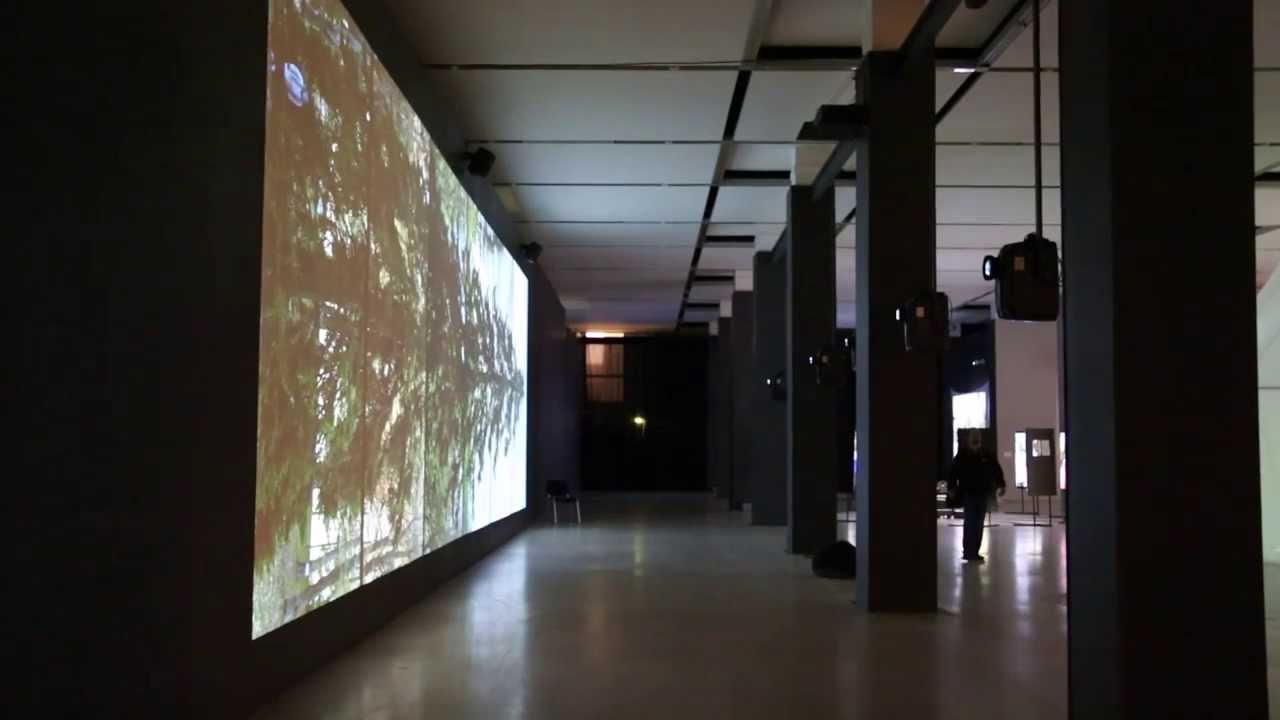This image depicts the interior of a dimly lit building, possibly a museum or exhibit hall, taken at night or when it's closed. The viewer looks down a long corridor framed by a series of black pillars on the right and a large multi-panel screen on the left. The ceiling is white with black and silver strips, providing faint illumination. Between the first three of the seven visible pillars, there are black projectors or lamps hanging down, casting a horizontal image of a tree with green branches and a white sky background onto the screen. The floor is made of shiny, bare concrete or marble. On the left side, a black chair is positioned against the wall near the screen. Further into the room, a person in dark clothing—possibly black shirt and blue jeans—walks towards the camera. The back wall appears to be gray or dark gray with a window outlined in black and covered with a white or tan shade, illuminated by a yellow light source. This room, with its stark contrast between black pillars and a white ceiling, creates a dramatic and eerie ambiance.